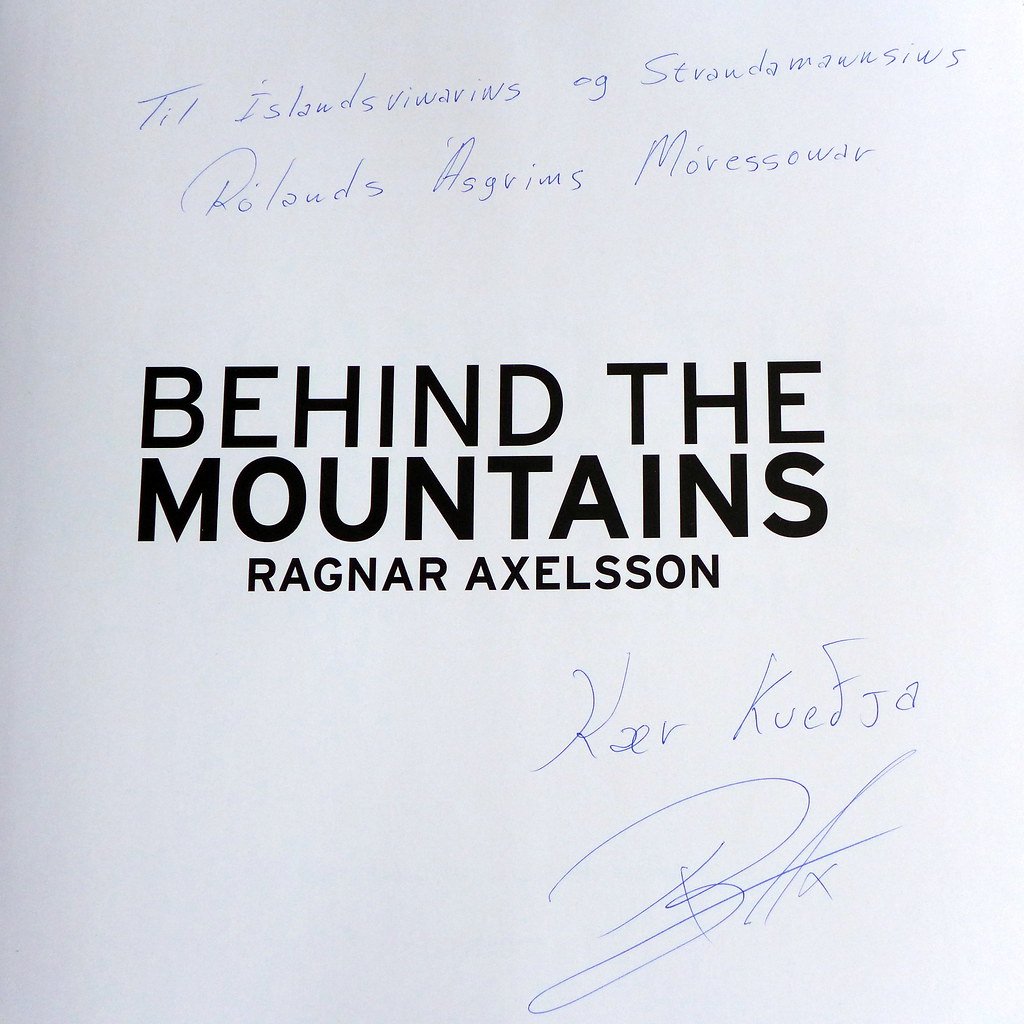The image displays a white piece of paper featuring a mix of printed and handwritten text set against a completely white background. Prominently, at the center of the paper, there is a bold, black-typed title that reads, "Behind the Mountains, Ragnar Axelsson." Spanning across the top of the image is a handwritten note listing names or words: "Till Islands, Vivians, OG, Stratamassus, Rolands, Aspim, More, Sober," though the exact transcription varies slightly. A signature accompanied by a possible handwritten note "Kur Kufja" appears in the bottom right corner. The colors present in the image are white, black, and blue. The overall composition suggests it may be a signed copy of a book title by the author.